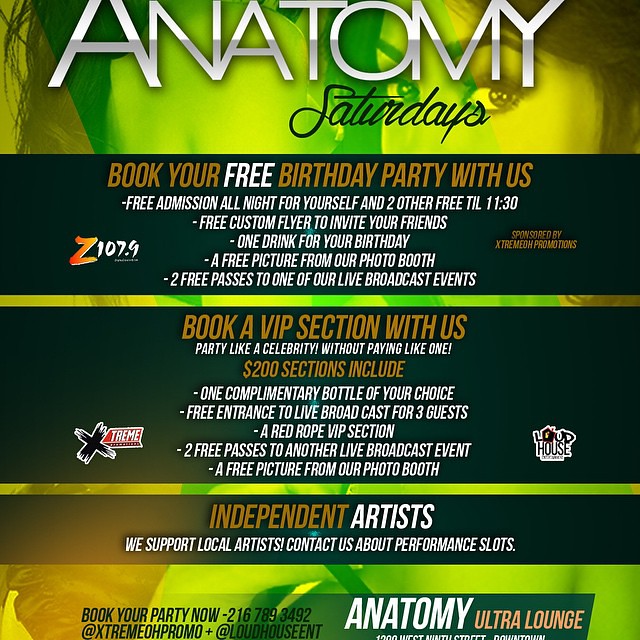**Anatomy Saturdays at Anatomy Ultra Lounge**

Join us for an unforgettable night with *Anatomy Saturdays*. Book your free birthday party with us and enjoy free admission all night for you and two guests until 11:30 PM. Receive a complimentary custom flyer to invite your friends, one free drink for the birthday guest, a free picture from our photo booth, and two free passes to one of our live broadcast events. Sponsored by Extreme Promotions and Z 107.9.

For a more exclusive experience, book a VIP section with us and party like a celebrity without the high cost. Our $200 VIP sections include one complimentary bottle of your choice, free entrance to live broadcasts for three guests, a red rope VIP section, two additional free passes to another live broadcast event, and another free picture from our photo booth.

We proudly support local independent artists. Contact us about performance slots and showcase your talent.

Book your party now at 216-789-3492. Visit Anatomy Ultra Lounge to celebrate your special occasions in style. Location details and further information are available upon request.